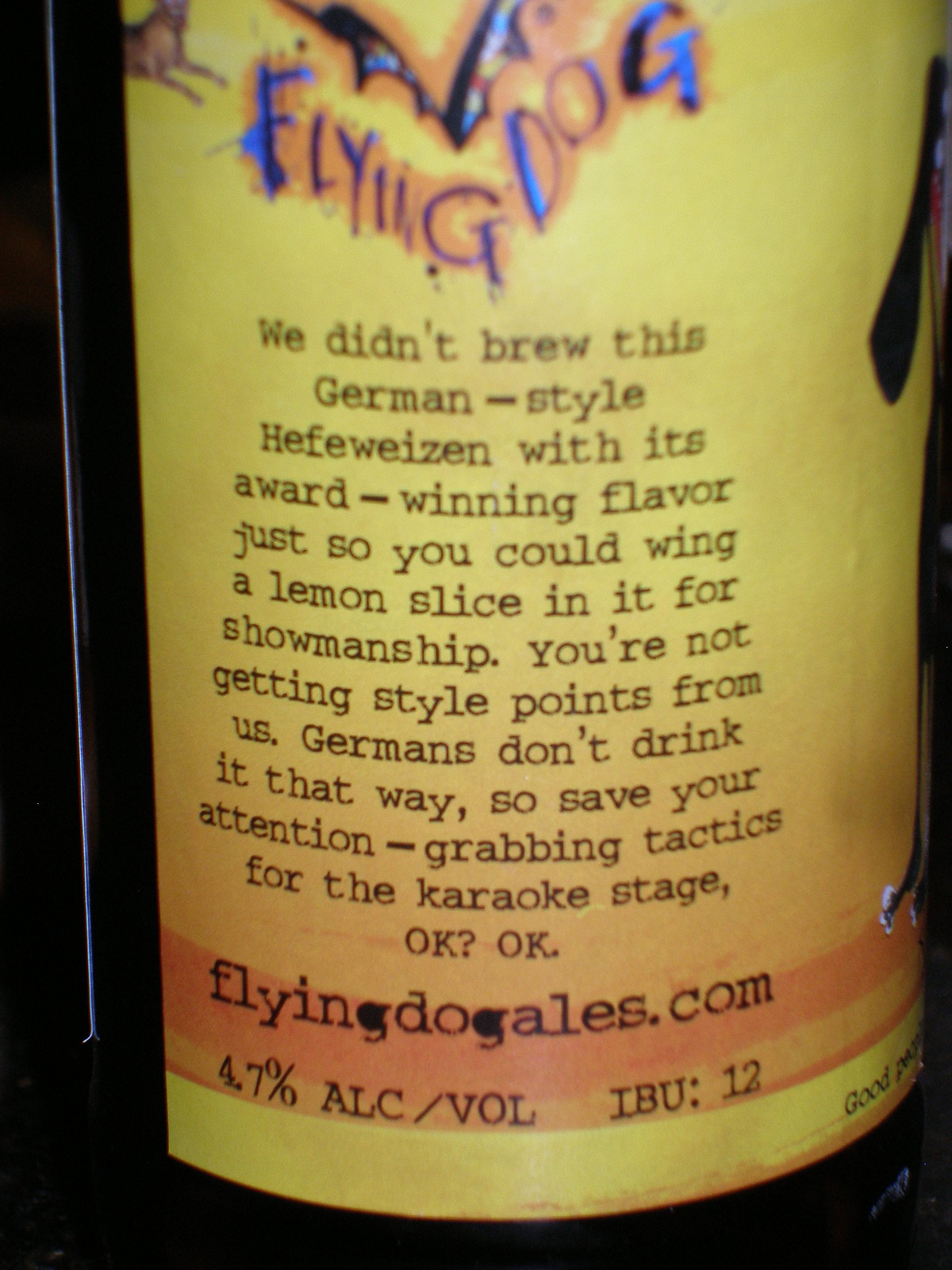The image captures a prominently displayed beer can in a dark setting, possibly a bar or dimly-lit room, with the background largely obscured. The can is adorned with a yellow label and takes center stage in the frame. At the top of the label, "Flying Dog" is written in dark blue, curved text outlined in orange, accompanied by an illustration of a flying dog with bat wings. Below the logo, a descriptive paragraph reads: "We didn't brew this German-style Hefeweizen with its award-winning flavor just so you could wing a lemon slice in it for showmanship. You're not getting style points from us. Germans don't drink it that way, so save your attention-grabbing tactics for the karaoke stage." This text is in black. Further down, the label includes the website "flyingdogales.com" and additional information about the beer's alcohol content (4.7%) and IBU, set against a slightly orange ribbon. The label also hints at other visual elements, such as a partially visible image of a dog to the left and a cut-off image of a woman to the right. The colors on the label include black, gray, yellow, brown, blue, and red, reflecting a vibrant yet sophisticated aesthetic.